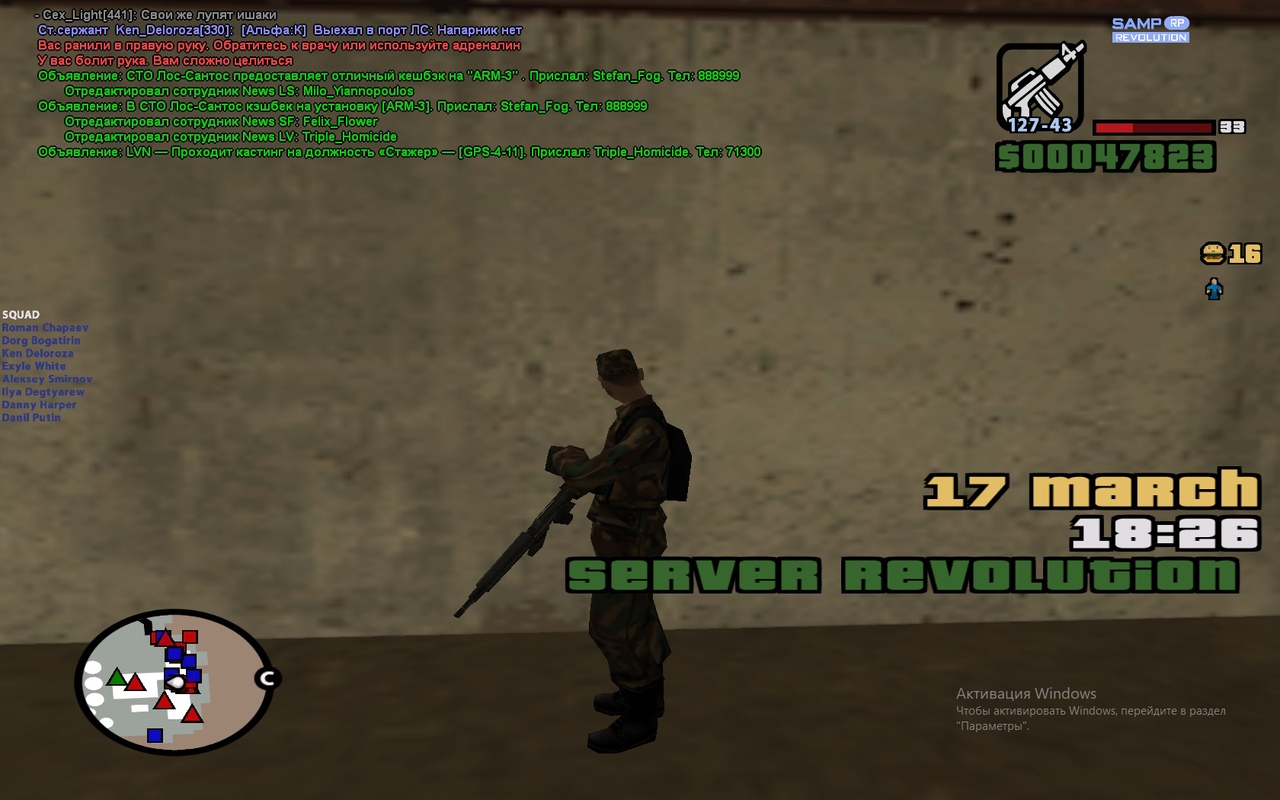This image is a screenshot from a video game, displaying a detailed user interface with a soldier as the main focus. The soldier, clad in camouflage attire and black boots, is holding a long rifle pointed diagonally to the left of the screen. His silhouette is highlighted against a tan background and a brown floor.

To the soldier's right is a block of text with various colors and borders: "17 March" in yellow with a black border, "18=26" in thick white text, and "server revolution" in green, also with a black border. Below this, there are several lines of text in what appears to be Russian, with the English word "windows" visible in gray. 

The lower left corner of the screen features a circular map, marked with different symbols including white rectangles, white circles, red triangles, and various squares, indicating the soldier's position relative to other objects and entities in the game. 

At the top of the screen, there are lines of green, blue, red, and gray text, likely corresponding to in-game chat or information. The upper right corner displays game stats, featuring a gun icon with the numbers 127-43, possibly indicating ammunition or score, alongside other metrics such as a status bar at 33, a price of 0 0 0 4 7 8 2 3, and the text "Sam RP Revolution". Additional elements include a burger icon with the number 16 and a small human figure.

The left side of the screen includes more text in various colors, providing details like the name of the squad, which includes members such as Roman Chapetdor, Alexei Smirnoff, Ilya, and others. The overall composition provides extensive information about the player's status, location, and objectives within the game.